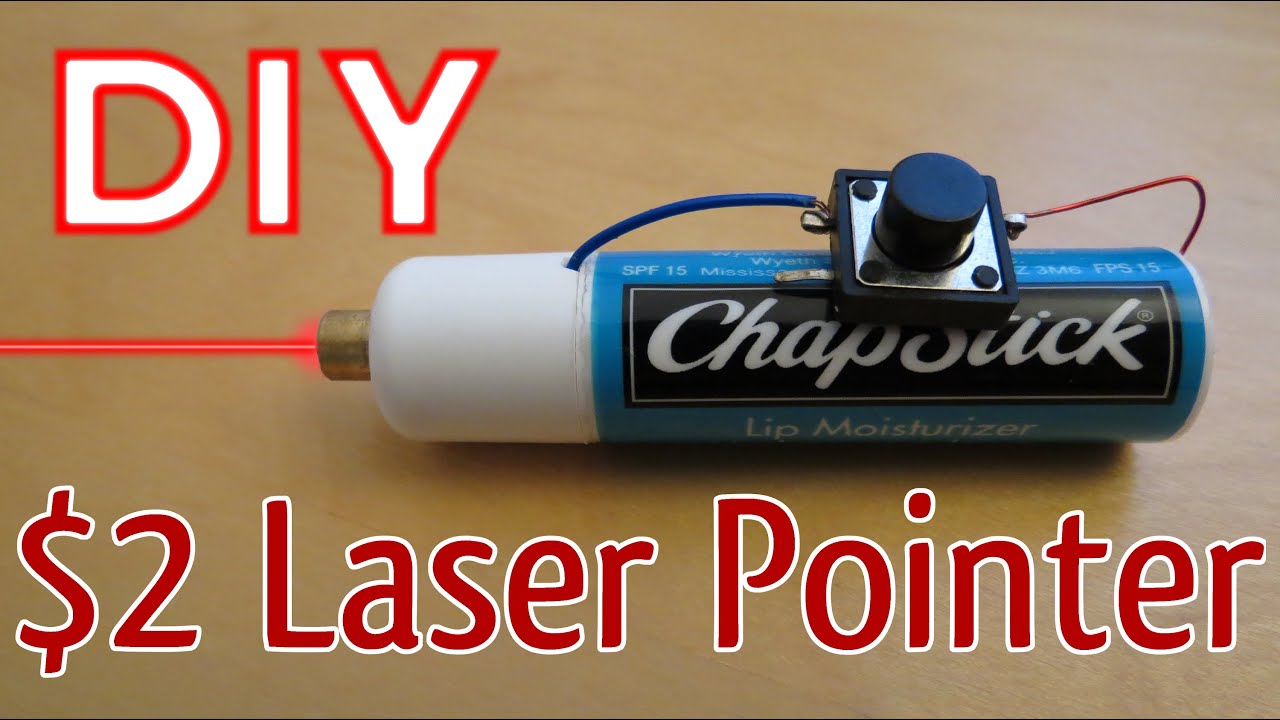This image showcases a do-it-yourself (DIY) $2 laser pointer project, prominently captioned with "DIY" in bold white letters with a red trim at the top left corner and "$2 laser pointer" in red letters with a white trim at the bottom. The DIY creation features a ChapStick container with a white lid, modified to emit a red laser through a small brass tip. The ChapStick tube itself is blue, marked with a black label stating "ChapStick" in white text, and "lip moisturizer" below it. 

The container has two holes on its side, through which red and blue wires run into the chapstick tube. These wires are connected to a small, square, silver metal switch with a blue button located at the center of the ChapStick casing. The entire setup is placed on a light brown wooden table, making the elements of this inventive laser pointer project clearly visible.